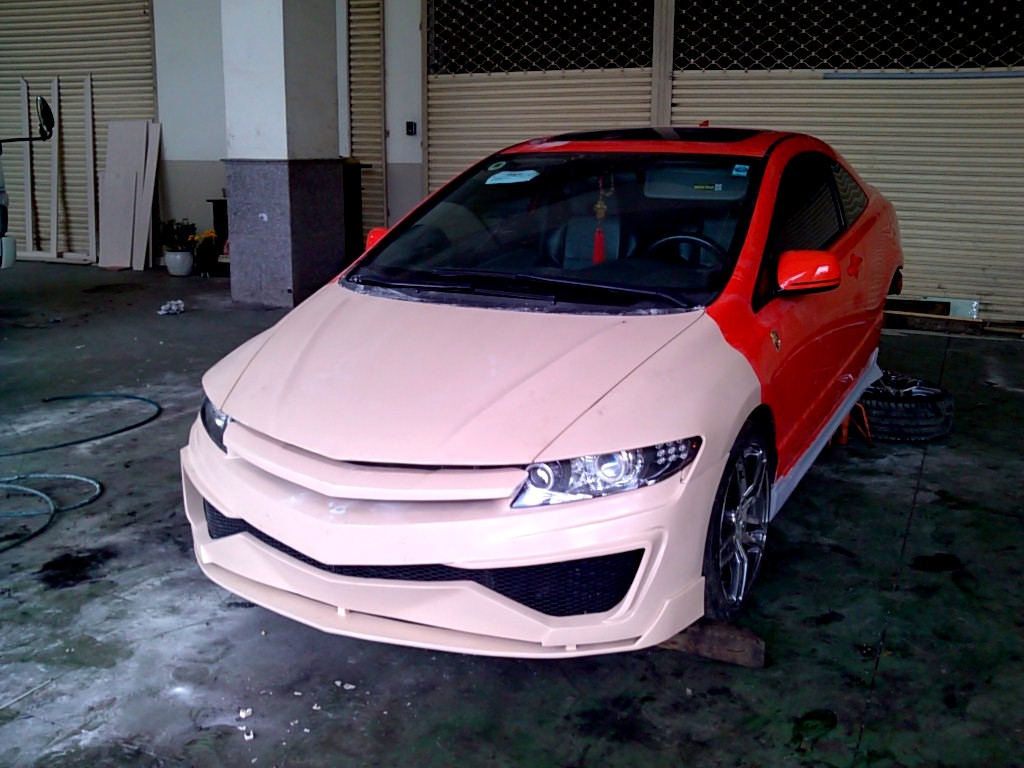In this image taken in a dimly lit car repair shop, a car is prominently featured against a metal-backed and concrete-floored garage. The vehicle, primarily red with a white front end, is parked adjacent to the garage door. The front of the car is slightly angled towards the lower left portion of the image. A distinctive white stripe runs along the bottom from the front wheel to the back. The car appears to be undergoing some form of repair, as the back wheel on the driver’s side is missing and lies flat on the ground next to the car. Through the window, you can see the driver’s side wheel interior. To the left of the vehicle, from the observer’s perspective, a green hose is clearly visible on the ground. The floor in the repair shop is strewn with various remnants of repair work, including fragments and whitish powder. There are no logos visible on the car, contributing to the ambiguity of its brand. The overall scene within the photograph has a somewhat dark ambiance, adding to the impression that the car, although parked near the garage door, is situated in an indoor space.